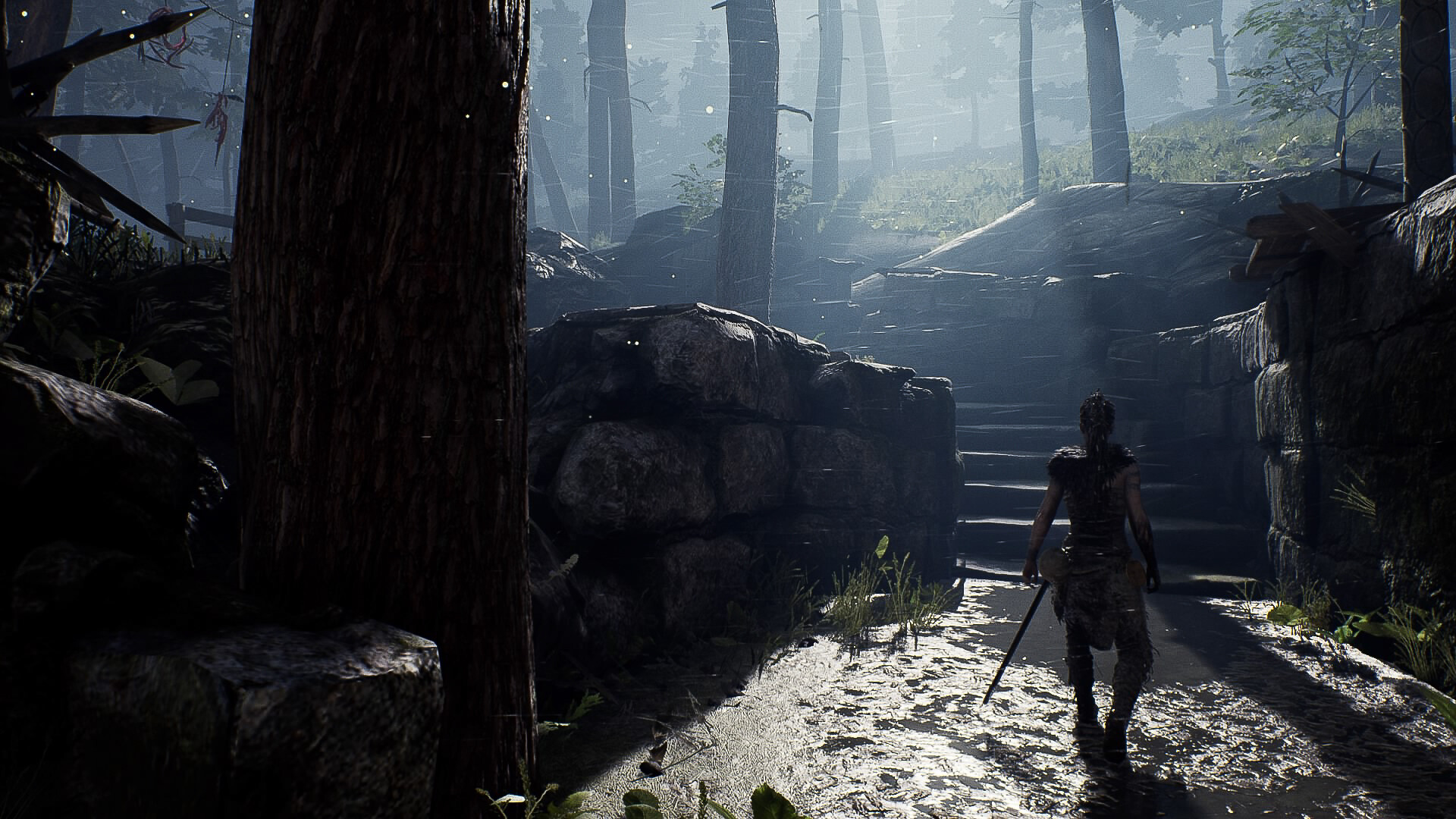The image appears to be a screenshot from a dark and atmospheric video game. Dominating the upper half of the image is a mist-shrouded forest, bathed in shades of gray, light gray, black, and green, creating a surreal and foggy ambiance. In the bottom right corner, a gray, rocky pavement can barely be made out due to the image's overall darkness. The silhouette of a lone figure—presumably a man—can be seen moving towards a staircase before him. His attire resembles that of a medieval warrior, featuring a skirt-like garment that reaches mid-thigh and a sword hanging from his left hip. A massive stone block wall runs parallel to him on his right, completely obscuring the top of the stairs in shadow. The same formidable stone wall extends to the left of the man, where it is joined by the base of a colossal tree trunk or pole that stretches from the bottom of the image all the way to the top, contributing to the ominous and foreboding atmosphere of the scene.